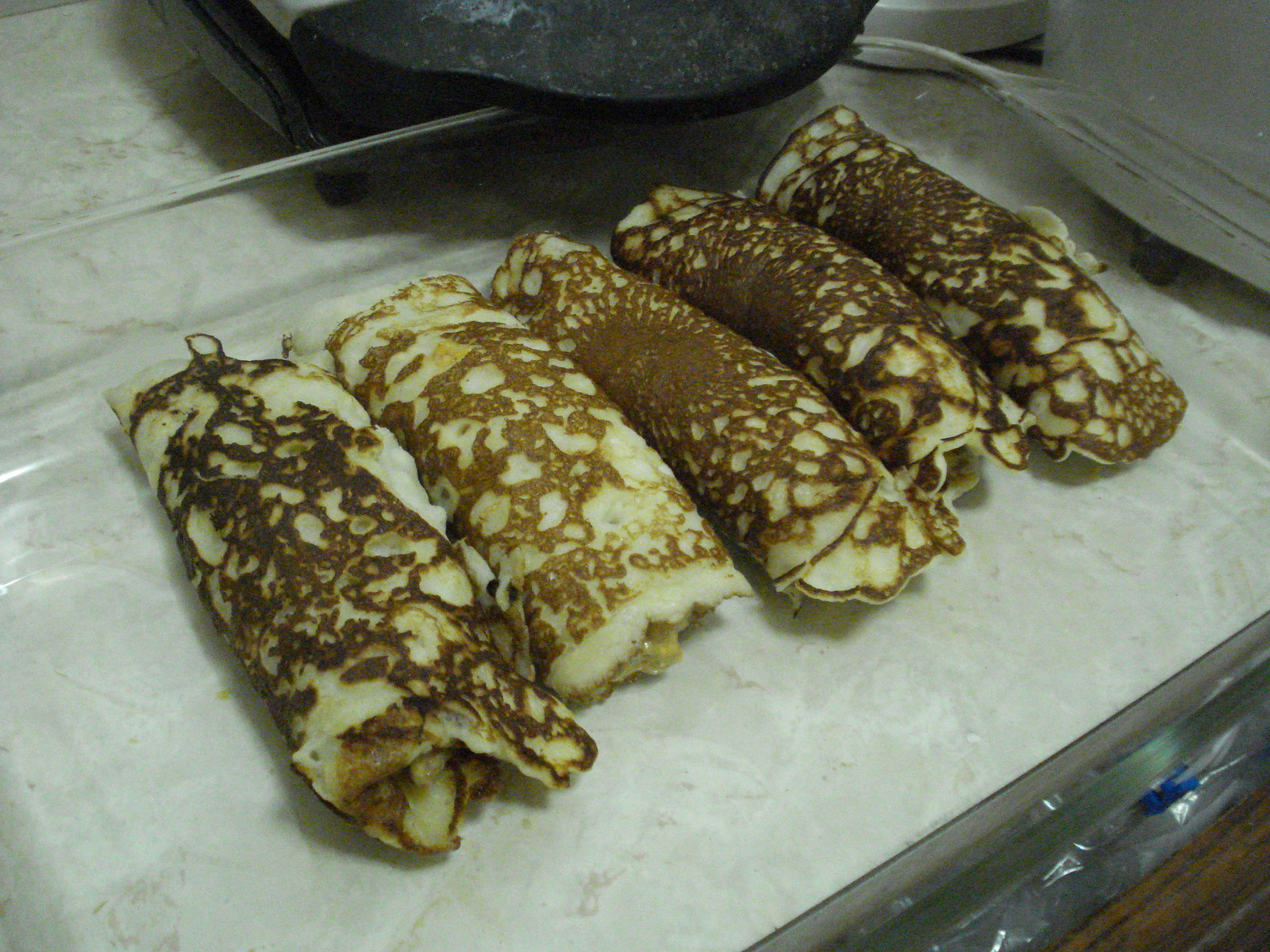This image is a detailed indoor color photograph taken under a bright flash, imparting a slight cyan tint. It depicts a large clear glass baking dish, likely a Pyrex, resting on a white Formica countertop. Inside the dish are several rolled pancakes or crepes arranged vertically against each other, creating a mesmerizing pattern of golden brown textures with hints of darker, almost burnt spots. Each roll is approximately seven inches long and three to four inches in diameter, aligned diagonally from the bottom left to the top right of the image. The crepes exhibit a toasted exterior, and some appear filled, with one roll possibly leaking a golden sauce or liquid. Surrounding the glass dish in the top middle and right portions of the image are various kitchen appliances or equipment, which are partially visible. The left side of the baking dish is slightly cut off, but the handle on the right side is clearly visible as a plain glass protrusion, set against what may be a marble or linoleum surface.